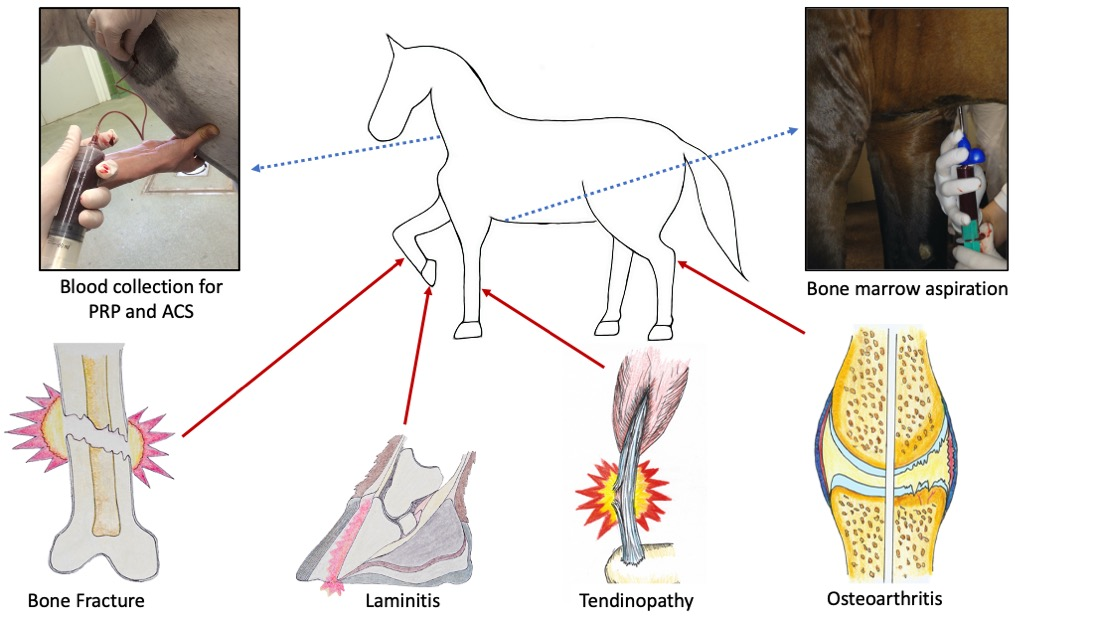The diagram provides a comprehensive overview of various equine leg health issues, featuring multiple visual elements against a white background. Central to the image is a line drawing of a horse, facing left, with its right front hoof raised. This drawing is connected by red arrows to a series of photographs and illustrations that detail specific medical conditions.

In the top left corner, a photograph labeled "Blood Collection for PRP and ACS" depicts a syringe withdrawing blood from a horse's neck area. Meanwhile, the top right corner features another photograph labeled "Bone Marrow Aspiration," showing a gloved veterinarian inserting a long hypodermic needle into the abdomen of a horse.

Below the central horse drawing, there are four labeled illustrations. The first, on the bottom left, depicts a broken bone split in the center, labeled "Bone Fracture," with an arrow pointing to the horse's raised front leg. Next to it, an illustration labeled "Laminitis" shows erosion on a horse's hoof, connected by an arrow to the raised hoof. Further to the right, an image labeled "Tendinopathy" portrays an inflamed tendon highlighted in red and yellow, with an arrow pointing to the supportive front leg on the ground. The final drawing on the bottom right, labeled "Osteoarthritis," shows a swollen, irregular joint, again marked with an arrow linking it to the horse's back leg.

Together, these visual and textual elements effectively illustrate significant equine leg health concerns such as bone fractures, laminitis, tendinopathy, and osteoarthritis, providing a clear and detailed educational resource.